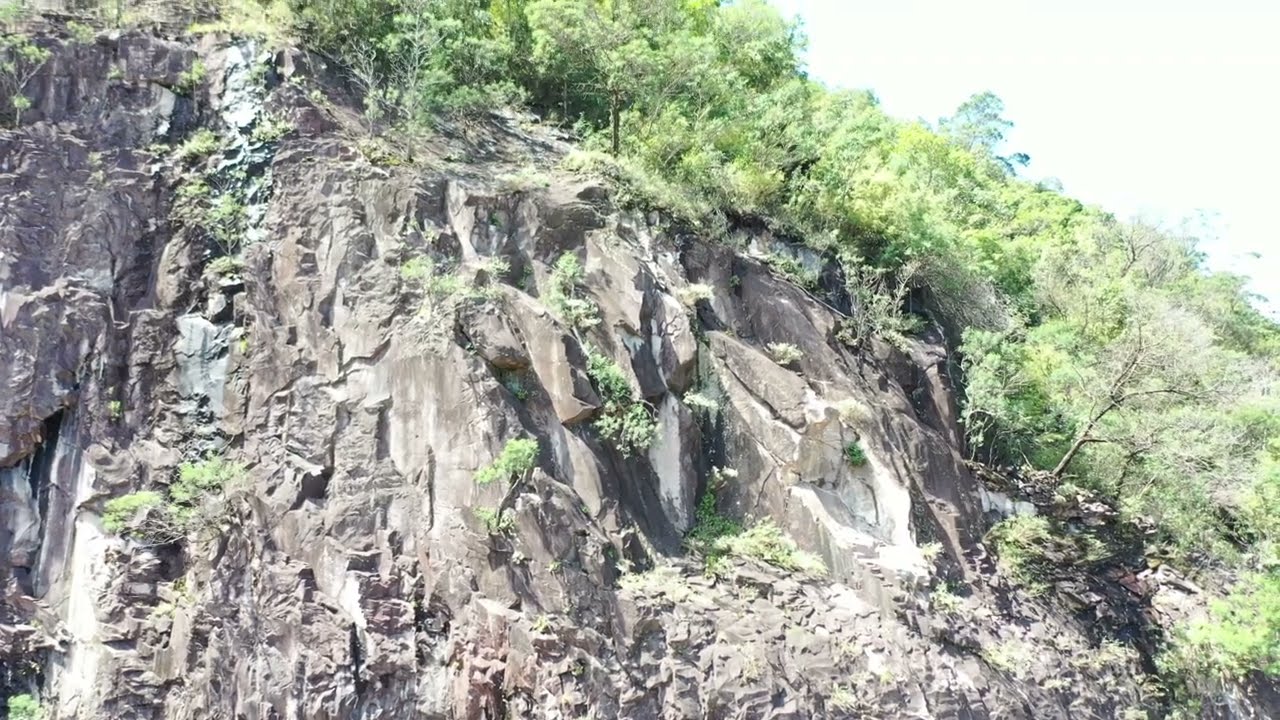The photograph captures a rugged granite cliff face dominating the left two-thirds of the image, with sharp, jagged edges and a light brown hue. The granite exhibits a nearly vertical ascent, interspersed with sparse but lush plant life, including young, skinny trees and various green bushes and grass sprouting from the rocky surface. Towards the right, the cliff slopes downward, where it is gradually enveloped by a dense cluster of trees showcasing a spectrum of greens—from lime to medium green—with some yellow highlights. These trees are more concentrated along the right side of the image, while at the top right, a small triangular patch of the sky peeks through, appearing exceptionally bright and white due to the sunlight beaming down, suggesting a clear sky. The overall scene suggests it is springtime, with the fresh, vibrant foliage contrasting against the stark, rocky granite.